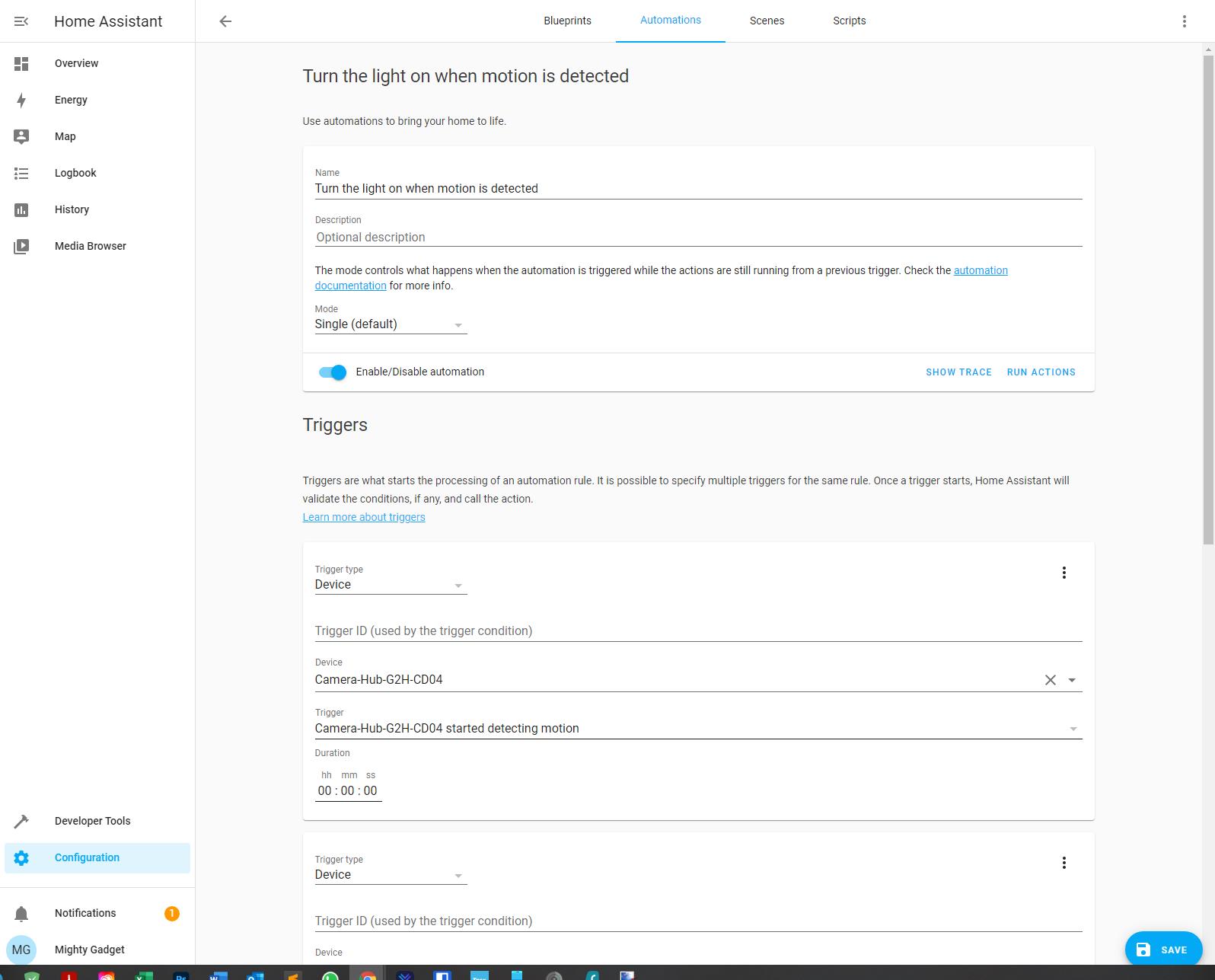The image depicts a Home Assistant dashboard displayed on a computer screen. On the left side, there is a vertical menu with options such as Overview, Energy, Map, Logbook, History, Media Browser, Developer Tools, and Configuration. The Configuration option is highlighted in blue and features a settings icon, indicating it is currently selected. Below these options, there is a section for Notifications and an entry labeled "Mighty Gadget."

At the bottom of the screen, the Dock for the computer is visible, while the top right corner of the screen displays tabs for Blueprints, Automation, Scenes, and Scripts. The Automation tab is highlighted in blue, suggesting it is the active section. On the main part of the screen, there is a prominent automation task titled "Turn the light on when motion is detected." Accompanying this title, a tagline reads, "Use Automations to bring your home to life."

Beneath the automation title, there is an optional description explaining that the mode controls what happens when the automation is triggered while actions from a previous trigger are still running. Additionally, there are sections for specifying triggers, devices, and cameras involved in the automation process, providing a comprehensive setup interface for managing a smart home.